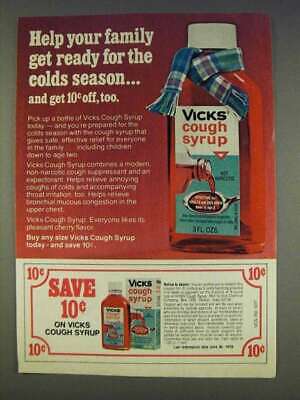This vintage Vicks Cough Syrup advertisement, likely from the 1970s, prominently features a bottle of the syrup wrapped in a plaid scarf, symbolizing warmth and protection during the cold season. Against a green background, the top half of the ad is strikingly red, drawing attention to the bold white letters in the top left-hand corner, which read: "Help your family get ready for the cold season and get 10 cents off too." The bottle, with its white cap and detailed label instructing how to pour the syrup into a spoon, is placed on the right side of the ad. The ad's bottom portion includes a white coupon outlined with red numbering, clearly stating, "Save 10 cents on Vicks Cough Syrup," amidst the vivid red and green hues that make this promotion eye-catching and memorable. The accompanying paragraph provides further details about the benefits of Vicks, ensuring families are well-prepared for the cold season.